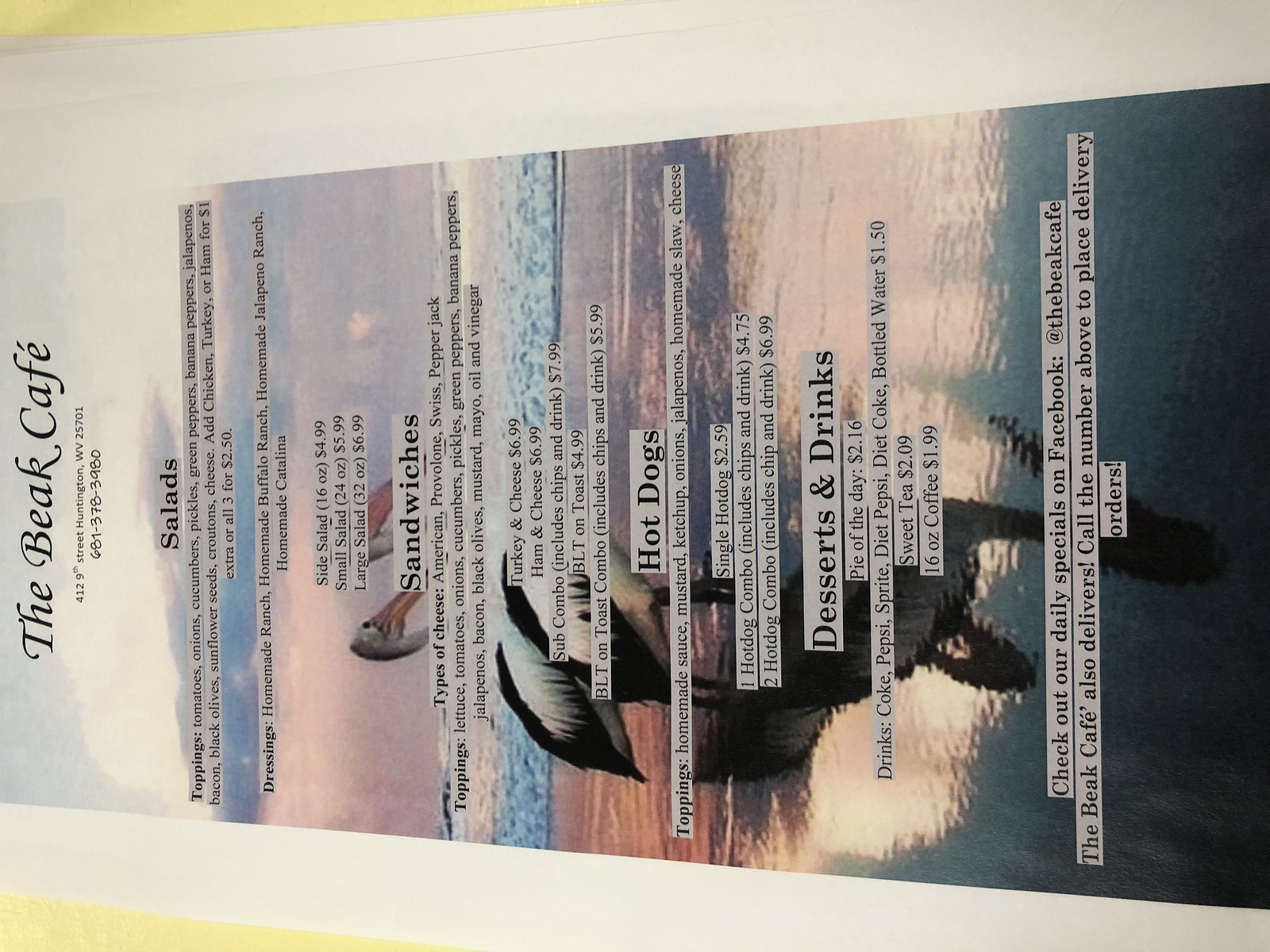This is an image of a menu for The Beak Cafe, although the image is displayed sideways, making it somewhat challenging to read. The menu prominently features the cafe's name and address, along with a contact number, which appears to be (687) 378-3980.

The menu starts with a section dedicated to salads, listing a variety of toppings such as tomatoes, onions, cucumbers, pickles, green peppers, and banana peppers. There are different salad sizes offered: a side salad, a small salad, and a large salad, each accompanied by two pricing options. Above this, a selection of dressings is displayed.

Following the salad section, the menu presents an array of sandwiches, detailing the types of cheese available and a list of toppings. There are also some specials or pre-made options like the turkey and cheese sandwich.

Next, the menu features hot dogs, including the available toppings. Options range from a single hot dog to two-hot dog servings, with a combo pack that includes chips and a drink.

At the bottom of the menu, there's a section for desserts and drinks. Additionally, the cafe advertises their social media presence, encouraging customers to check out their daily specials on Facebook.